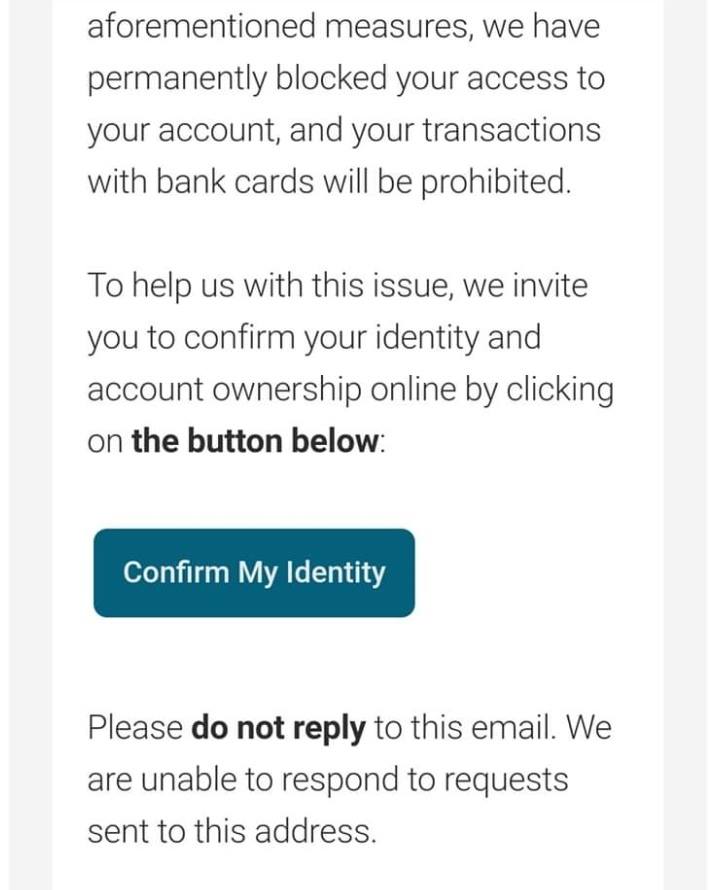This image is a screenshot from a website or app, featuring a fraud alert or warning message concerning account activity. The message is displayed on a white background with vertical gray dividers on both sides, suggesting a formal layout often used in emails. 

The first paragraph, written in black text, states: "Aforementioned measures we have permanently blocked your access to your account and your transactions with bank cards will be prohibited." This clearly indicates that the user's account has been blocked and any transactions using their bank cards will not be processed.

The second paragraph urges the user to confirm their identity to address the issue: "To help us with this issue, we invite you to confirm your identity and account ownership online by clicking on the button below." Below this paragraph, there is a prominent button labeled "Confirm Identity" in white text on a dark aqua blue background.

Following the button, there is a third paragraph in bold that advises: "Please do not reply." It further explains, "Please do not reply to this email. We are unable to respond to requests sent to this address."

Overall, the image appears to capture a critical alert, most likely a fraud notification, informing the user of blocked access and requesting them to confirm their identity through the provided link.